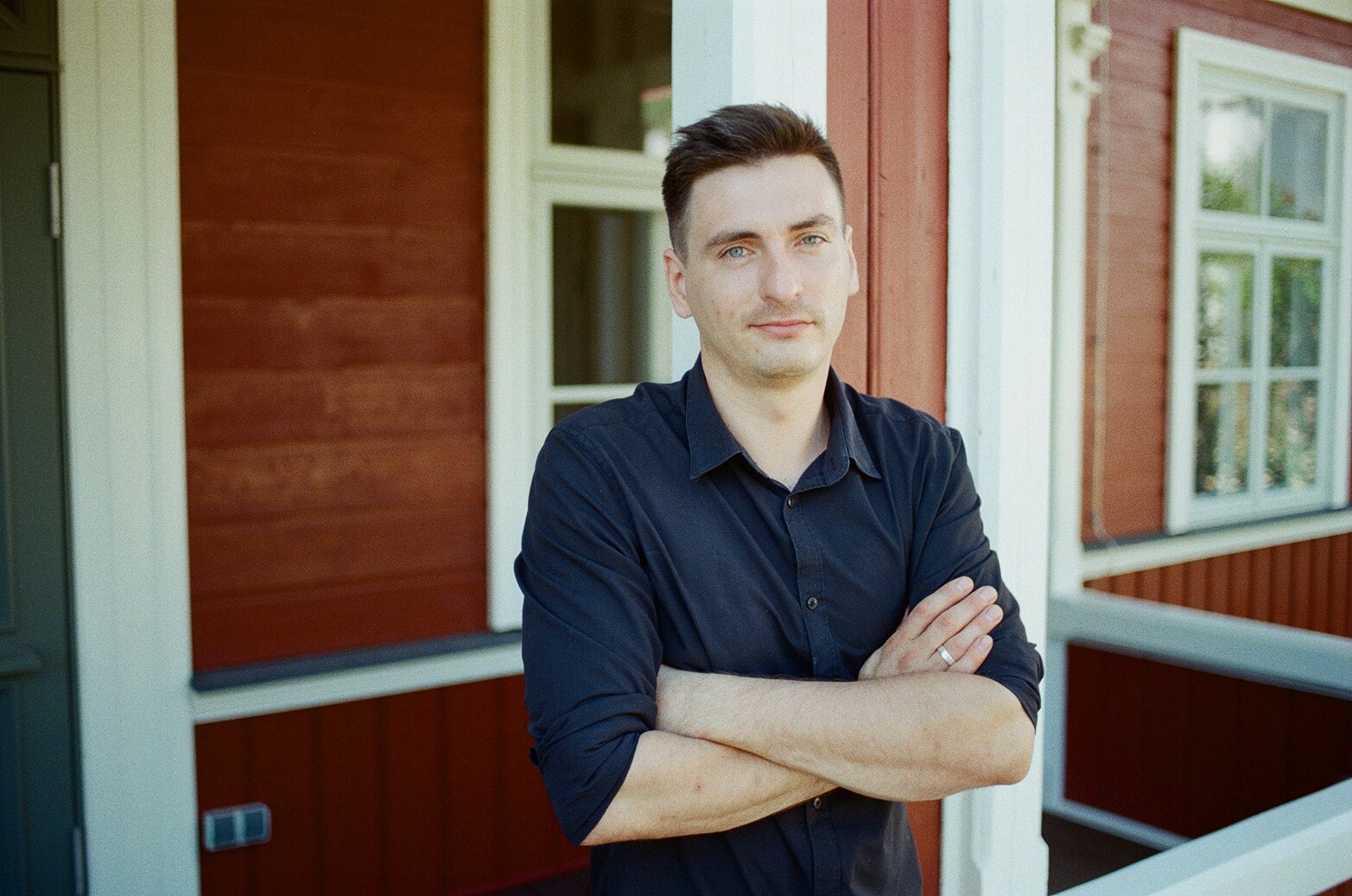The photograph depicts a man standing outside of a red house with white window frames. The man, who is white with short hair styled in a pompadour cut, appears to have a slight smirk or a Mona Lisa-esque smile on his face, suggesting mild amusement or reluctance at being photographed. He has light blue eyes, with hints of green, and his features include a 5 o'clock shadow and a shaven mustache. He is dressed in a blue button-up shirt, with the sleeves rolled up, and has a gold ring on his right ring finger. The house behind him, painted with a brick-like red hue and adorned with white shutters, serves as a picturesque backdrop to his casually crossed arms pose on the porch.